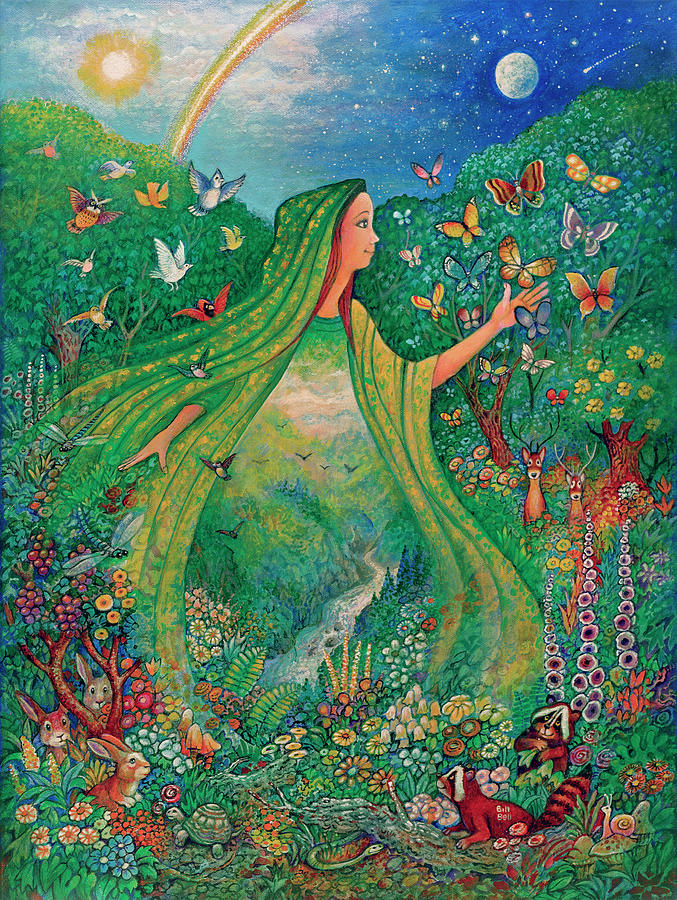This hand-drawn, colorful illustration could easily serve as the cover of a greeting card. It prominently features a young woman with shoulder-length red hair, donned in a green cloak with a hood that seamlessly blends into the natural setting around her, almost like a personification of Mother Nature. The scene is vibrant and lively, with her dress transforming into a landscape that includes a meandering stream, mountains, flowers, and lush trees. The background is split into a dazzling sun with a rainbow on one side, and a night sky with a moon and shooting stars on the other, symbolizing a harmonious blend of day and night.

Surrounding the central figure, the environment is teeming with life: colorful butterflies in hues of red, orange, yellow, black, pink, and blue flit around the trees, while numerous birds in corresponding shades soar above. At her feet, a host of small animals including rabbits, squirrels, raccoons, and a turtle gazing up at her add to the scene's enchanting quality. In the background, a couple of deer can be seen among the flora. The woman has her hands extended in a gesture of nurturing, enhancing the overall feel of harmony and the thriving, bustling nature around her.